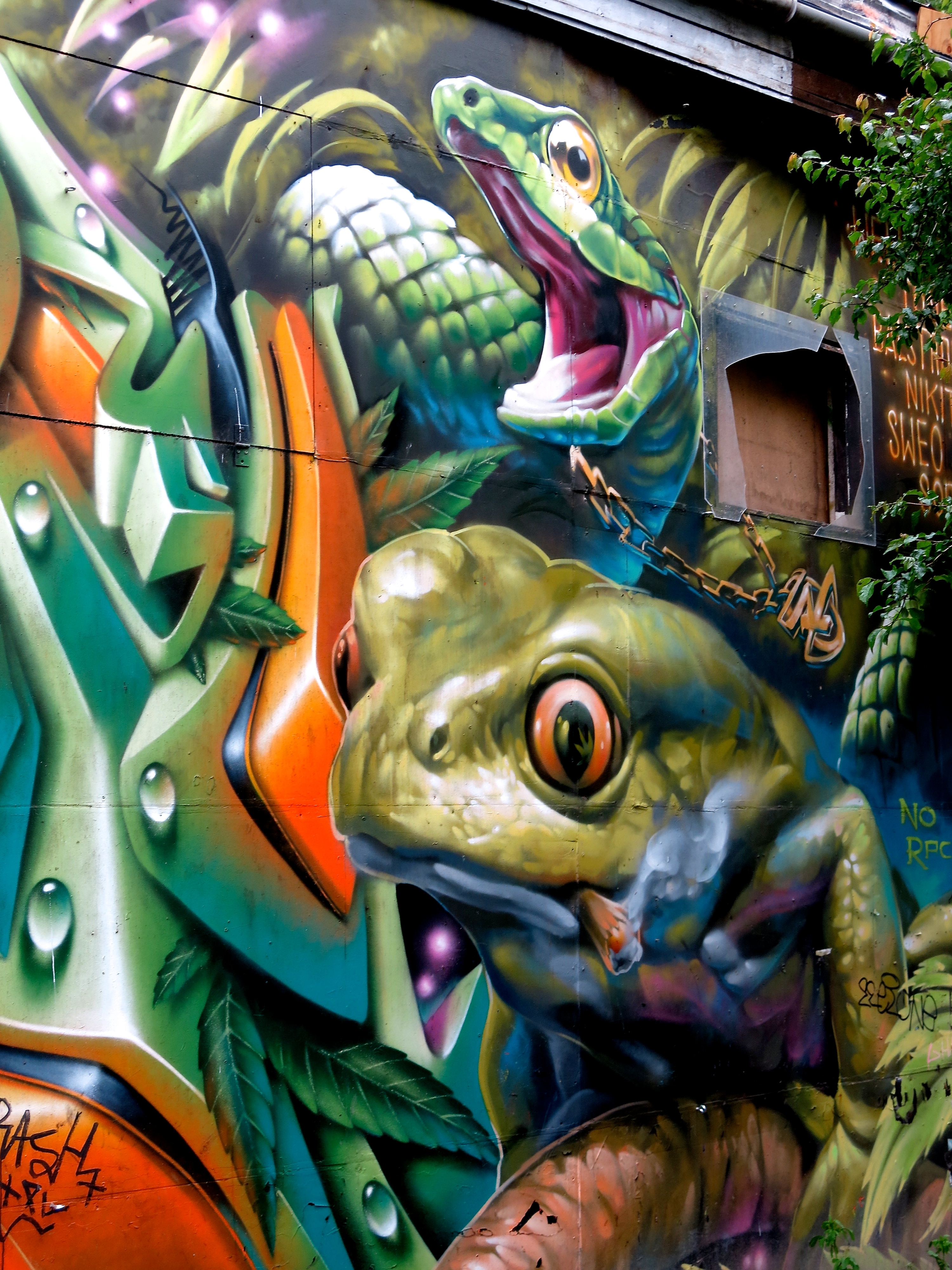This detailed mural, painted on the side of a house, features a vibrant, animated frog and a fierce green snake. The frog, perched on a curved tree branch, sports a colorful design with lime green on the top, pinkish-orange eyes, and a blue and purple underbody accented with yellow. A whimsical touch is added by the cigar in its mouth, with smoke curling upwards. Adjacent to the frog, the green, scaly snake stands out with its bright pink open mouth, giving it a ferocious appearance as though it's ready to bite. 

The mural is rich with decorative elements: on the left, a curved orange pattern adorned with small crosses and the letters "A-S-H" in black, surrounded by green and white pearls. Surrounding the creatures, the background features modern machinery in shades of green, blue, and orange, and on the right, a partially cut-off tree and an illegible sign next to what appears to be a broken window or vent. This imaginative and colorful scene creates a captivating visual story on the wall.